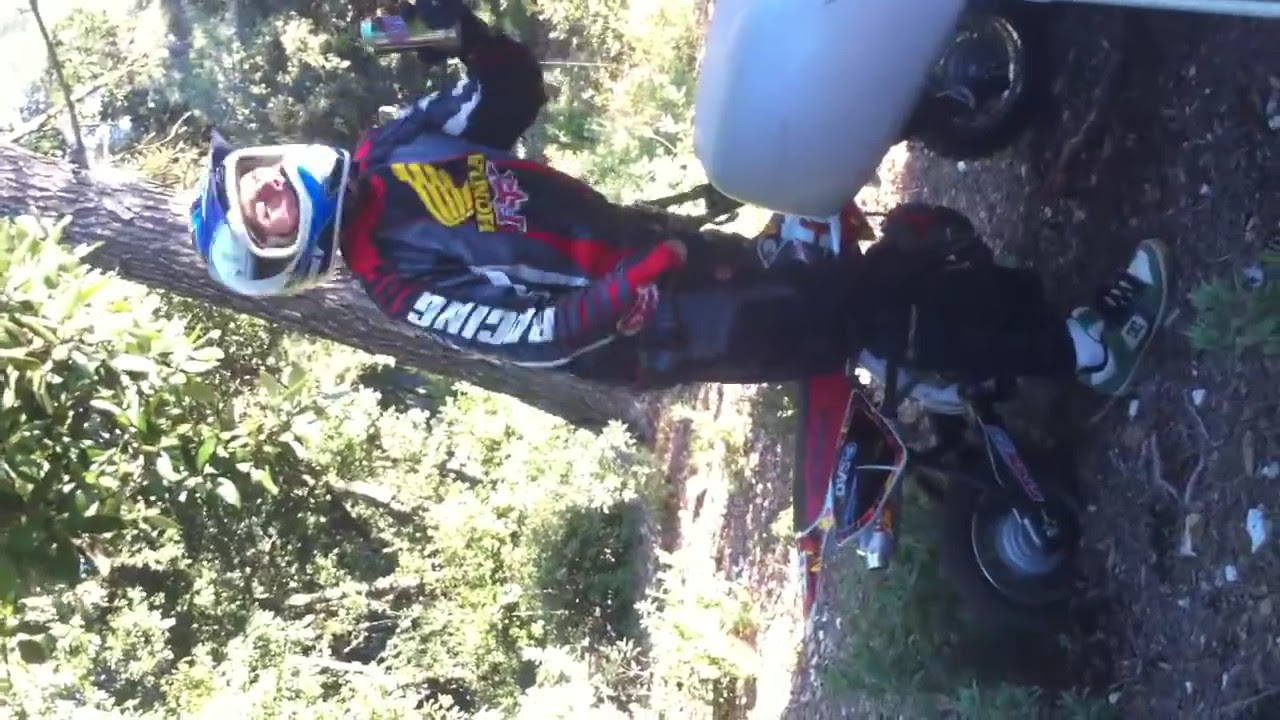In the brightly lit outdoor setting of a park or garden, a man stands the focal point of the photograph, which is tilted 90 degrees counterclockwise. Dressed in dark racing gear, the suit features various insignias, including the word "Racing" on the sleeve and the Honda logo emblazoned in both English and Asian characters. His helmet, primarily white with royal and navy blue accents, complements the outfit. Although the man appears to be a biker or perhaps a race car driver, he is oddly perched over a tiny, child-sized red bike with a white section, adding a humorous twist to the scene. His green sneakers with black laces and a white "H" logo and his white socks are visible. The man's left hand holds a can, while his right hand rests at his side. The ground beneath him is scattered with sticks, leaves, and white debris, further emphasizing the outdoor environment. Behind him, a tree with its trunk, branches, and green leaves is bathed in bright sunlight, enhancing the lively ambiance of the photo.